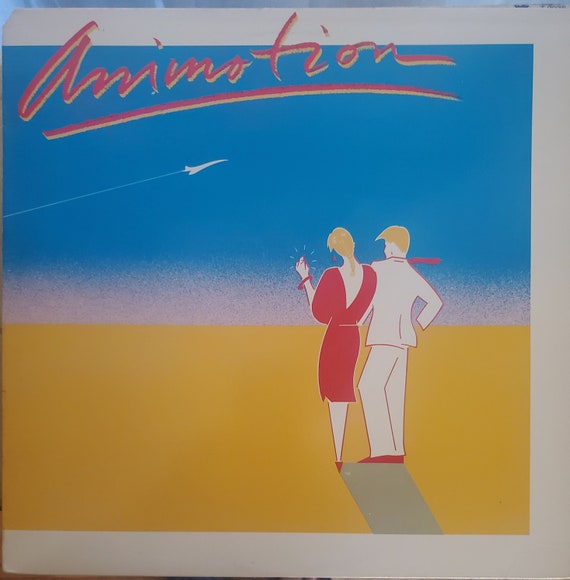The image is a detailed illustration with a square shape, measuring approximately four inches by four inches. It features a thin blue border at the very top, with subtle hints of gray. Enclosing the image is a light gray outer border about a quarter to half an inch wide, which descends from the top, down the right side, and across the bottom.

Inside this border, the background transitions from a golden yellow at the bottom, to a light pink strip, and finally into a blue sky at the top. Prominently displayed in red cursive letters, outlined in yellow, is the word "Animotion" at the top of the image. The cursive text extends partly beyond the borders, adding a three-dimensional effect.

In the foreground, a man and woman with blonde hair stand side by side, seemingly hand-in-hand. The woman, positioned on the left, wears a red dress, while the man, to her right, is dressed in a white suit accented with a red neckerchief and matching red shoes. Both characters have fair skin, contributing to a color palette dominated by white, red, and yellow.

Above them in the blue sky, there is a simple, white outline of a jet plane, resembling a Concorde, with a trail line extending behind it. The composition of the illustration gives a slightly abstract impression, with the characters gazing towards the plane, creating a sense of wonder and anticipation.